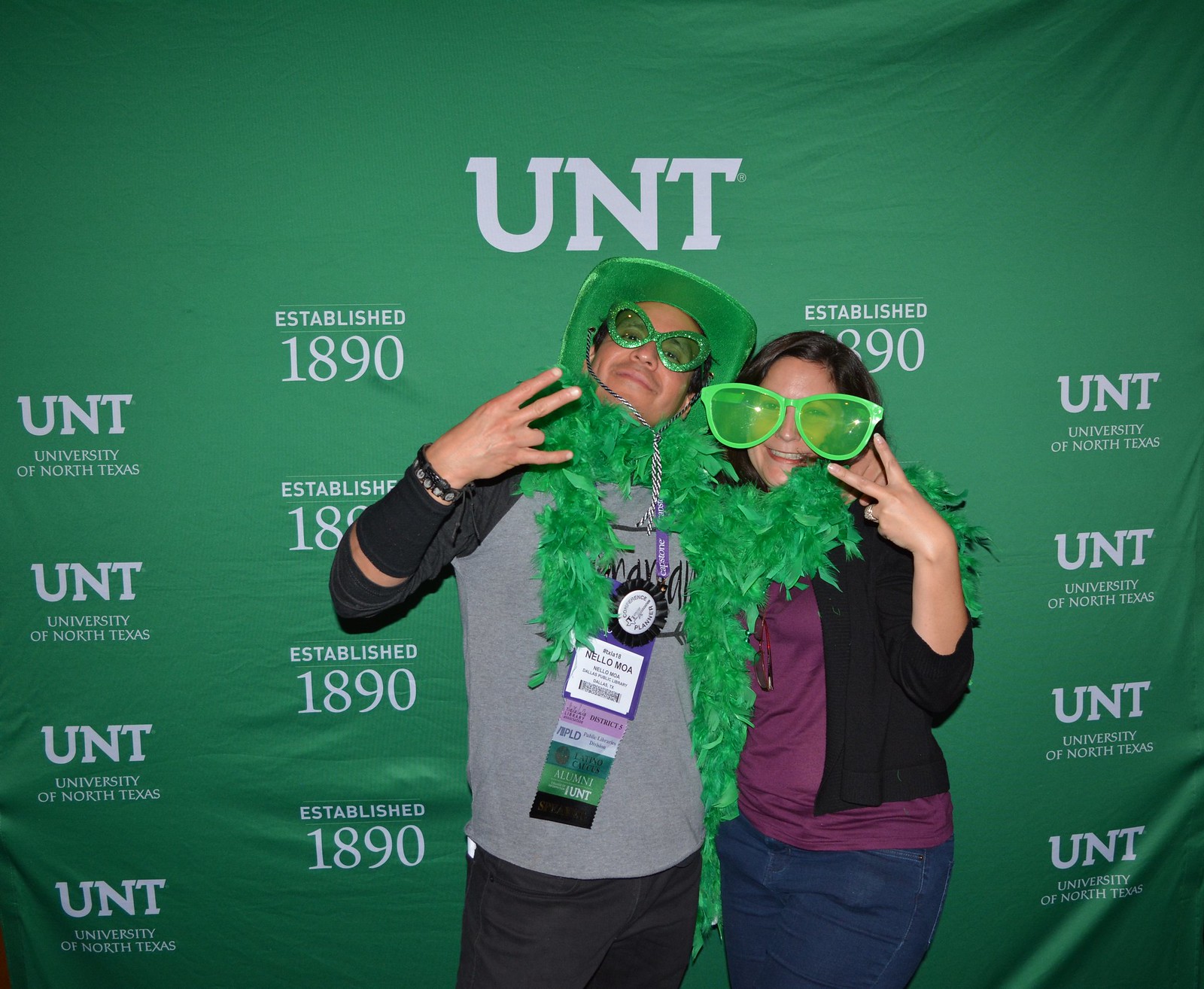A young couple, a man and a woman, smile brightly at the camera while standing against a vibrant green banner that prominently displays "UNT," "University of North Texas," and "Established 1890." The couple is clearly dressed to celebrate a UNT event, possibly a conference, as indicated by their festive attire. The man is wearing a gray T-shirt, shorts, a flamboyant green cowboy hat, and oversized sparkly green glasses. He also has a lanyard around his neck that reads "Nilo Moa, Dallas Public Library, Dallas, Texas, District 5 Public Libraries Division, Latino Caucus Alumni, Conference Planner." The woman complements his getup with a purple T-shirt, a sweater, jeans, and matching oversized green glasses. Both are adorned with a shared fluffy green scarf, and she is seen flashing a peace sign while he holds up three fingers with one bent. Additionally, she has a ring on her left hand, hinting at a special relationship between them. Their playful, spirited outfits and the repetitive UNT signage in the background tie them unmistakably to the University of North Texas celebration.